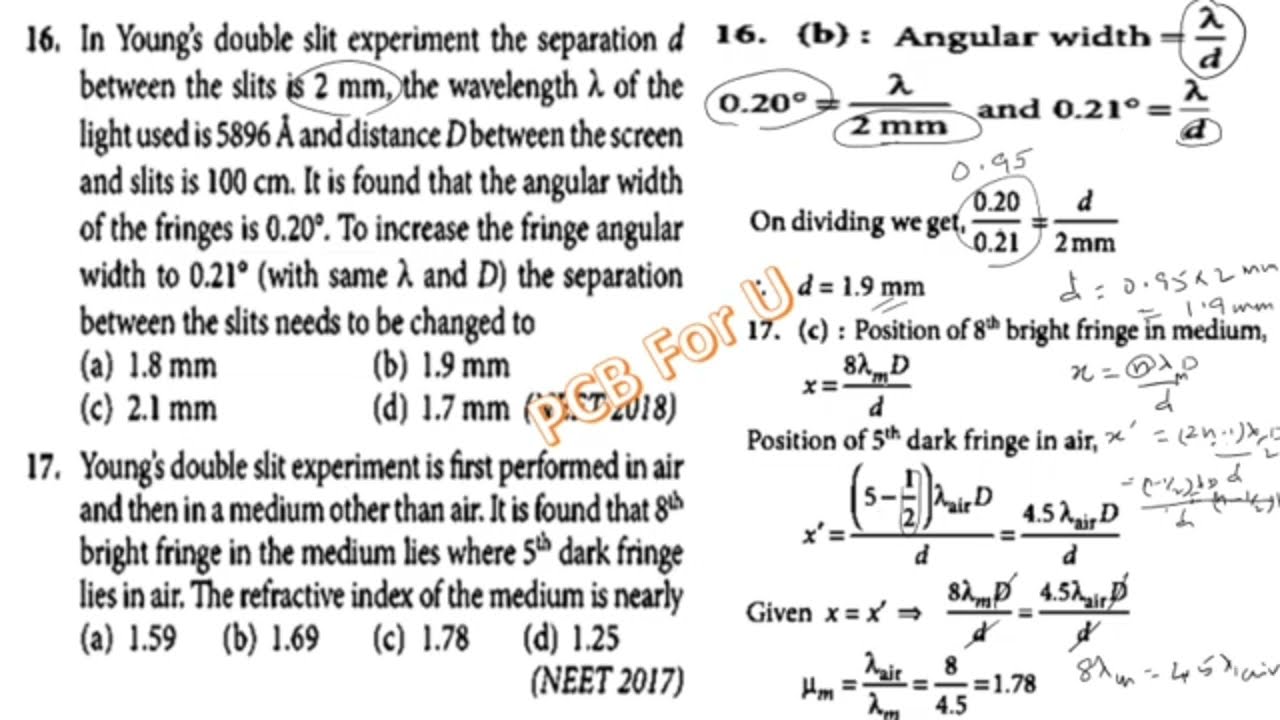The image features a mathematical word problem likely extracted from a test, with two numbered questions, 16 and 17, each accompanied by multiple-choice answers. The left side of the image contains the detailed text of these problems. Question 16 pertains to Young's double slit experiment, specifying conditions like a 2mm slit separation, a wavelength of 5896 Å, and a 100cm distance between the slits and the screen, with the problem aiming to determine the new slit separation required to achieve a specific fringe angular width of 0.2 degrees from various options (1.8mm, 1.9mm, 2.1mm, 1.7mm). Question 17 also revolves around Young's double slit experiment, this time comparing results in air and another medium to find the refractive index of the medium, with options (1.5, 1.69, 1.78, 1.25). The right side of the image presents two columns of text where the left column appears to restate part of the questions, while the right column comprises complex mathematical equations and calculations, including handwritten notes and circled figures, demonstrating iterative scratch work. This scratch work includes equalities and ratios pertinent to solving the given problems. A prominent watermark labeled "PCB4U" overlays the image.